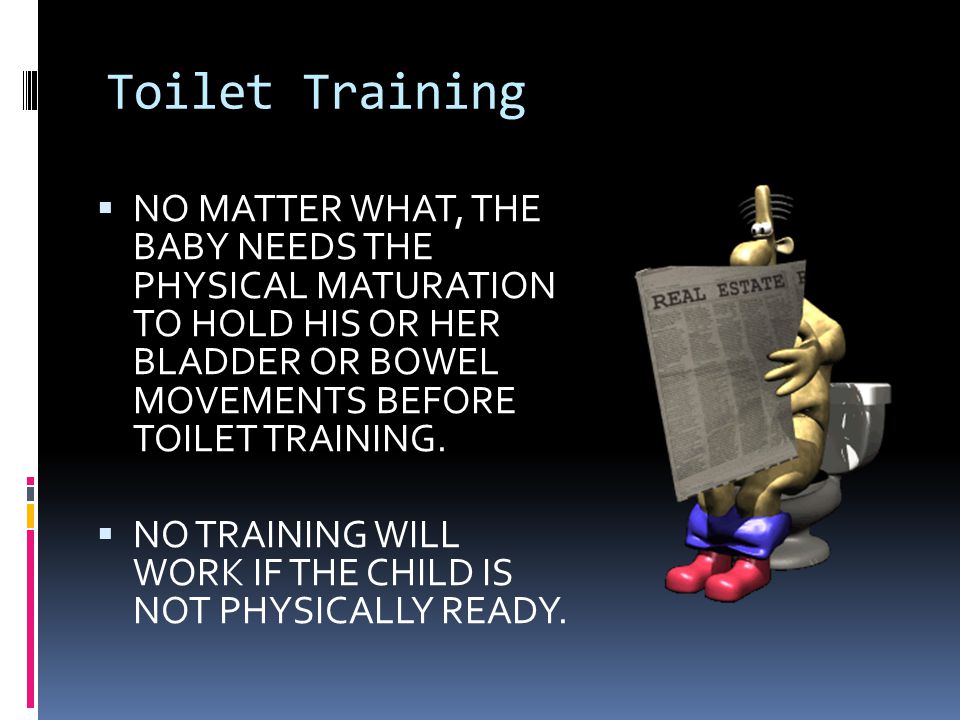The image features a black background that transitions into a lighter blue towards the bottom, creating an ombre effect. On the left side of the image, white text reads "Toilet Training," followed by two bullet points: "No matter what, the baby needs the physical maturation to hold his or her bladder or bowel movements before toilet training," and "NO TRAINING WILL WORK IF THE CHILD IS NOT PHYSICALLY READY," with the latter point emphasized in all capital letters. On the right side, a cartoon-like, digitally created yellow figure with eyes, a large nose, and three fingers is depicted sitting on a white toilet. The figure, which is humanoid in form but lacks a human head, is holding a newspaper labeled "Real Estate." The blue pants of the figure are rolled down to reveal red shoes at the base. The scene has a playful, illustrative quality, suggesting it is part of a PowerPoint presentation aimed at discussing the prerequisites for effective toilet training. The color scheme includes black, dark blue, light blue, gray, yellow, blue, red, and pink.